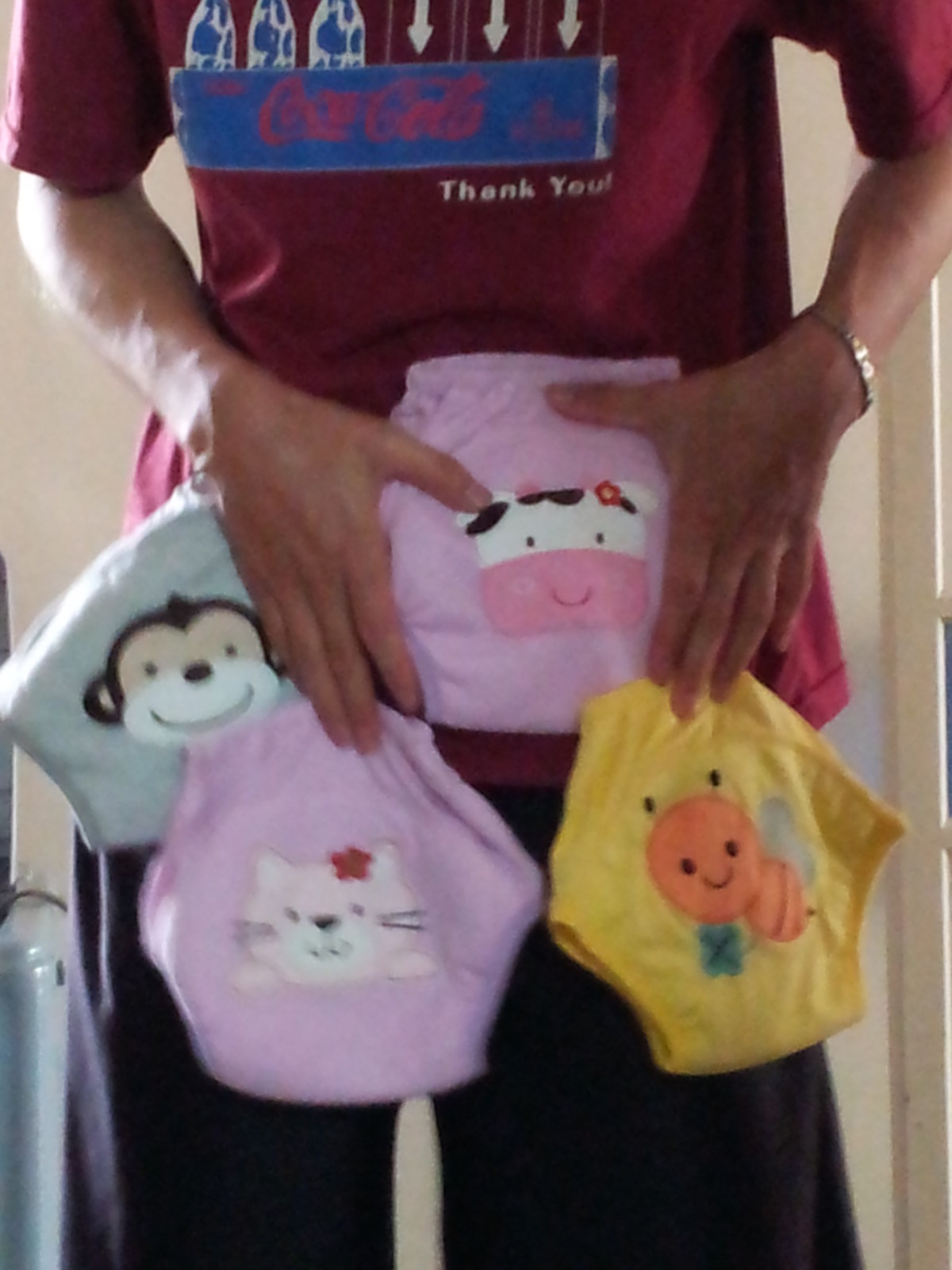A person is seen from the chest down, standing and facing the camera, wearing a dark burgundy shirt adorned with a Coca-Cola logo in red letters on a blue background. Above the logo are three downward-facing white arrows followed by three other symbols. In the corner underneath the logo, "thank you!" is written in white letters. The individual is wearing a thin gold bracelet on their left wrist. They are holding several children's cloth diapers in front of their stomach. The diapers include a pink one with a smiling cow featuring small dot eyes and a red flower on the left side of its head, a yellow one with an orange bee that has a green leaf and white wings, another pink one featuring a cartoon cat with a red flower on its left ear, and a blue one displaying a smiling monkey with a small button nose. The diapers are pentagon-shaped with sleeves at the top and leg holes at the bottom left and right.